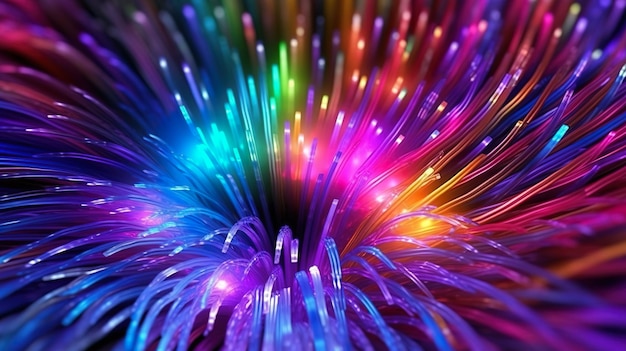The image displays a mesmerizing close-up view reminiscent of fiber optic cables or plastic filaments, radiating an explosion of luminous colors against a black background. The scene is dominated by a vivid array of colors including shades of blue, green, pink, purple, yellow, orange, and red. From a central point, these long, thin, glowing strands splay outward, creating an effect similar to a firework bursting in the night sky. The bright tips of the strands, particularly abundant in blue towards the bottom of the photograph, contribute to an intense light that gradually diminishes as it extends outward, while the vibrant colors continue to captivate the viewer with their brilliance.